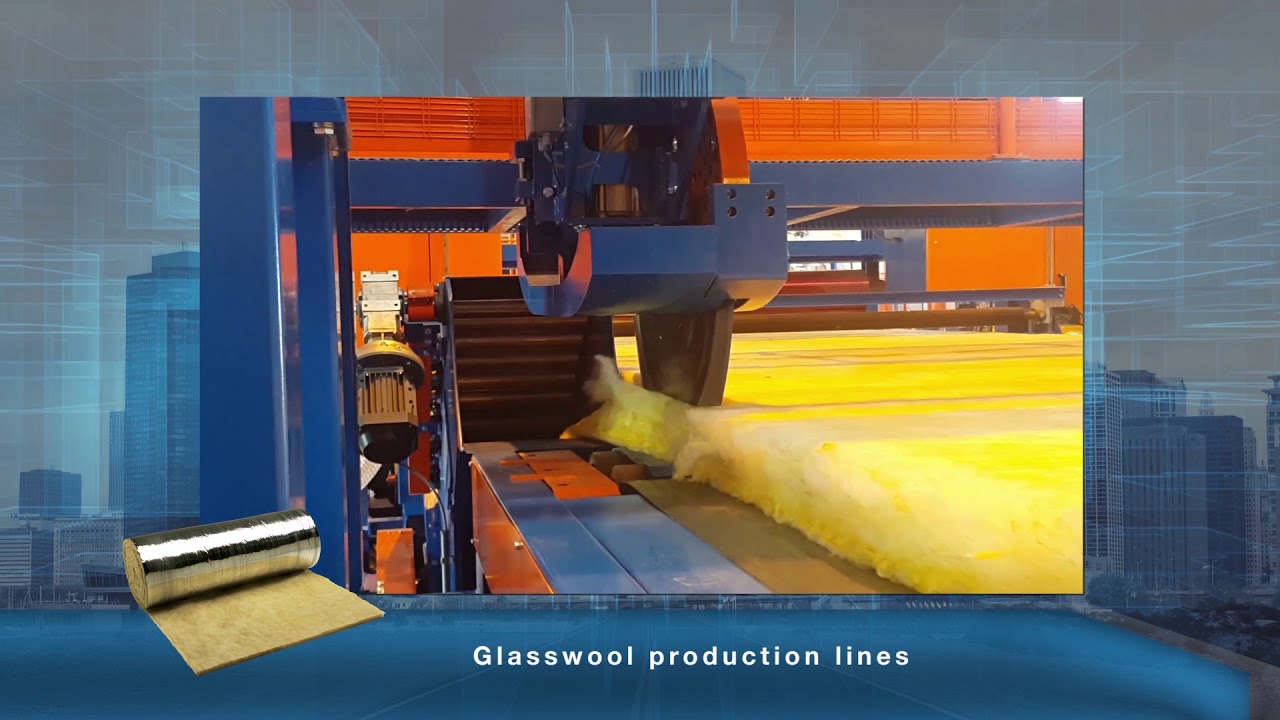The image is an industrial advertisement showcasing a glass wool production line. At the center, a large, blue cutting machine with a black circular saw is prominently displayed, cutting through yellow fiberglass batting. The batting has a shiny, metallic aluminum foil backing, visible in both the cut section and the large rolled section depicted. The machine operates on blue horizontal and vertical beams, set against an orange background that accentuates the blue machinery and the bright yellow fiberglass. Additional visual elements include a blurred digital background with blue and light brown cityscape tones. The edges of the image are framed in blue, with white text at the bottom stating, "glass wool production lines." The image appears to be part of a digital or print advertisement aimed at promoting industrial equipment for fiberglass production.